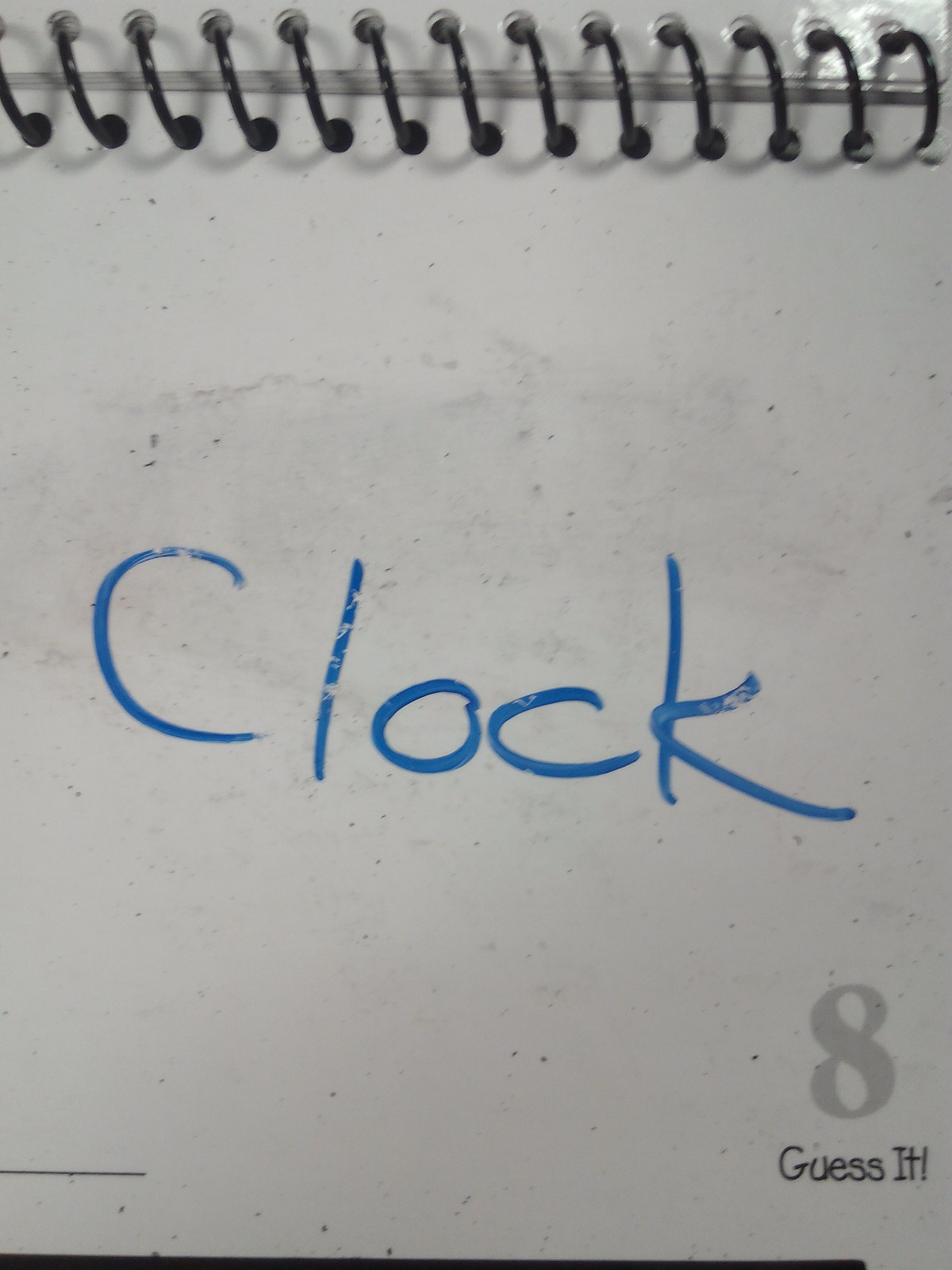The image is a vertically-oriented, first-person POV photograph of a unique dry erase notebook. The notebook has a spiral binding at the top, with visible holes from the spiral rings. The main focus is on the word "clock," written prominently in blue dry erase marker in the center of the whiteboard-like page, which shows signs of erasure and black splotches scattered across its surface, indicative of previous markings. In the lower right-hand corner, an engraved, sizeable gray number "8" is present, with the phrase "guess it!" etched below it in smaller font. There's also a faint horizontal black line emanating from the lower left corner, not extending all the way across the page. This intriguing image captures the blend of a traditional notebook's structure with a dry erase functionality, making it an unusual and eye-catching subject.